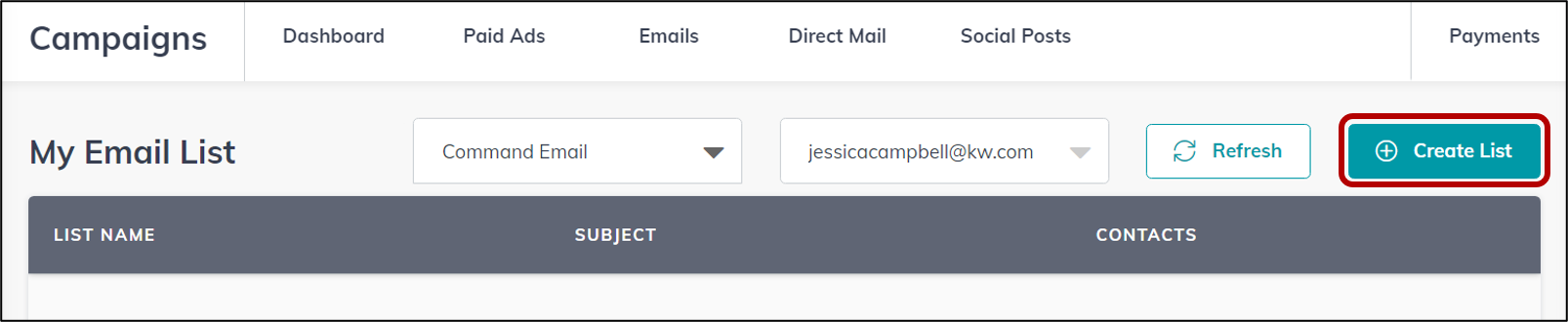The image features a white border at the top, within which various category labels are displayed in black text. Starting from the left, the labels read: "Campaigns," "Dashboard," "Paid Ads," "Emails," "Direct Mail," "Social Posts," and finally, in the top right corner, a smaller label "Payments."

Beneath this header, the background transitions to gray. On the far left side, in larger black text, the image displays the title "My Email List." Adjacent to this title is a horizontal white rectangle containing the text "Command Email" with a drop-down arrow on its right side. Next to it is another white rectangle filled with the text "Jessica Campbell at kw.com," which also features a drop-down arrow.

To the right of these rectangles, there is a smaller white rectangle with a circular icon made up of two arrows forming a loop, accompanied by the text "Refresh." Sitting to the right of this is a blue rectangle bordered in red, containing the text "Create List." To its left, there is a white circle featuring a white plus sign inside it.

Below these elements is a black banner that spans the width of the image. On the far left of this banner, in white text, it reads "List Name." Centered in the middle is the text "Subject," and aligned to the far right is the text "Contacts."